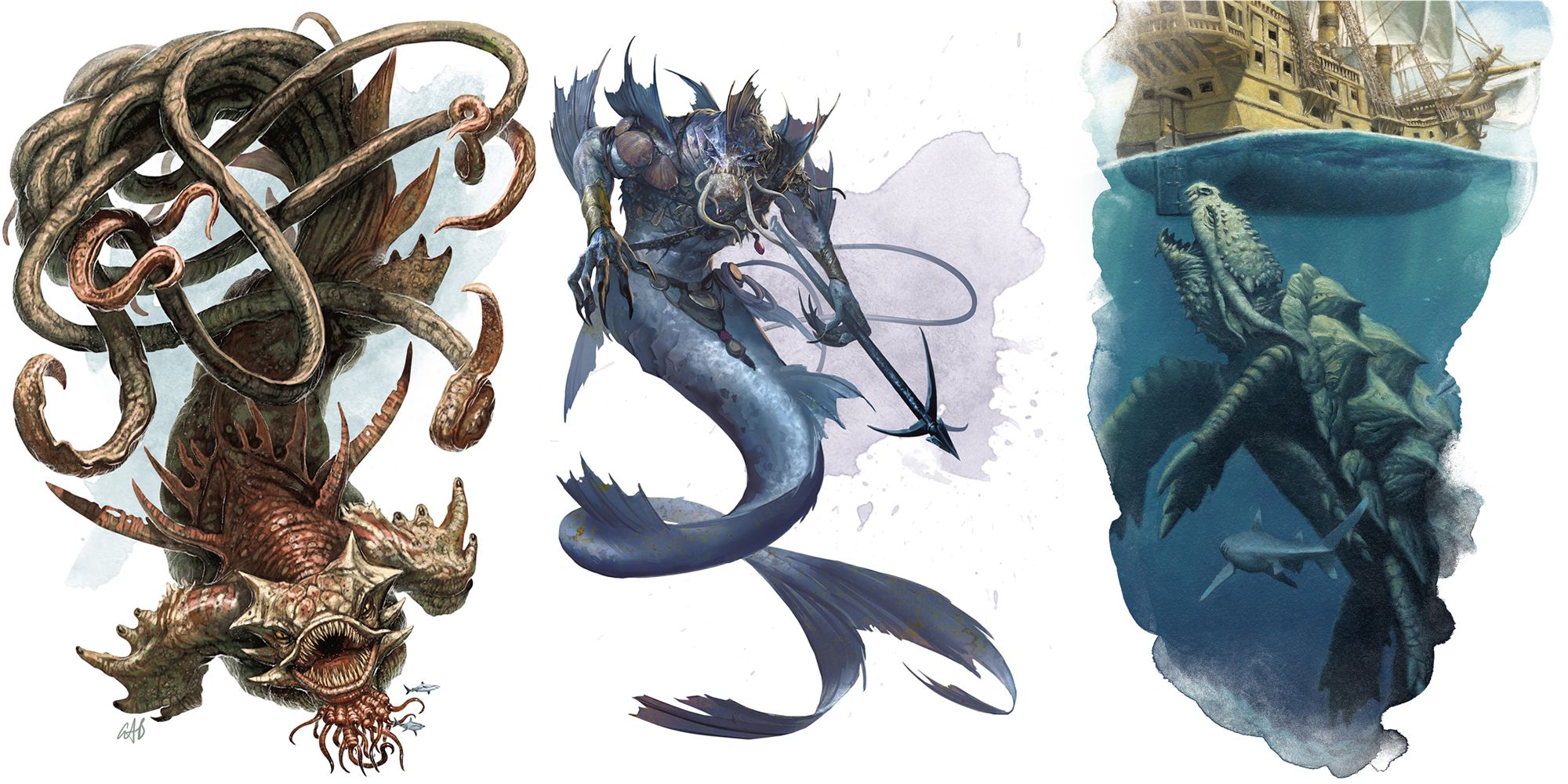The image showcases three distinct and detailed depictions of mythical water creatures, each separated vertically. On the left, there is a gigantic, piranha-faced fish monster with a reddish-orange hue. This menacing creature has large, arm-like fins and a lower body that splits into numerous thick, tentacle-like appendages. The middle section features a formidable merman-like being with a blue hue, brandishing a harpoon in its left hand. This creature has a mermaid tail that is long and curved, and is adorned with menacing claws, armor, and facial tentacles where a mustache might be. Finally, on the right, the image presents an ancient, colossal tortoise emerging from the water, seemingly poised to bite a boat floating above. This imposing turtle dwarfs a nearby shark, emphasizing its immense size and strength. The intricate details suggest the artwork is either a part of a video game or a fan-created drawing, with each creature rendering a vivid and fantastical exploration of mythical underwater beings.